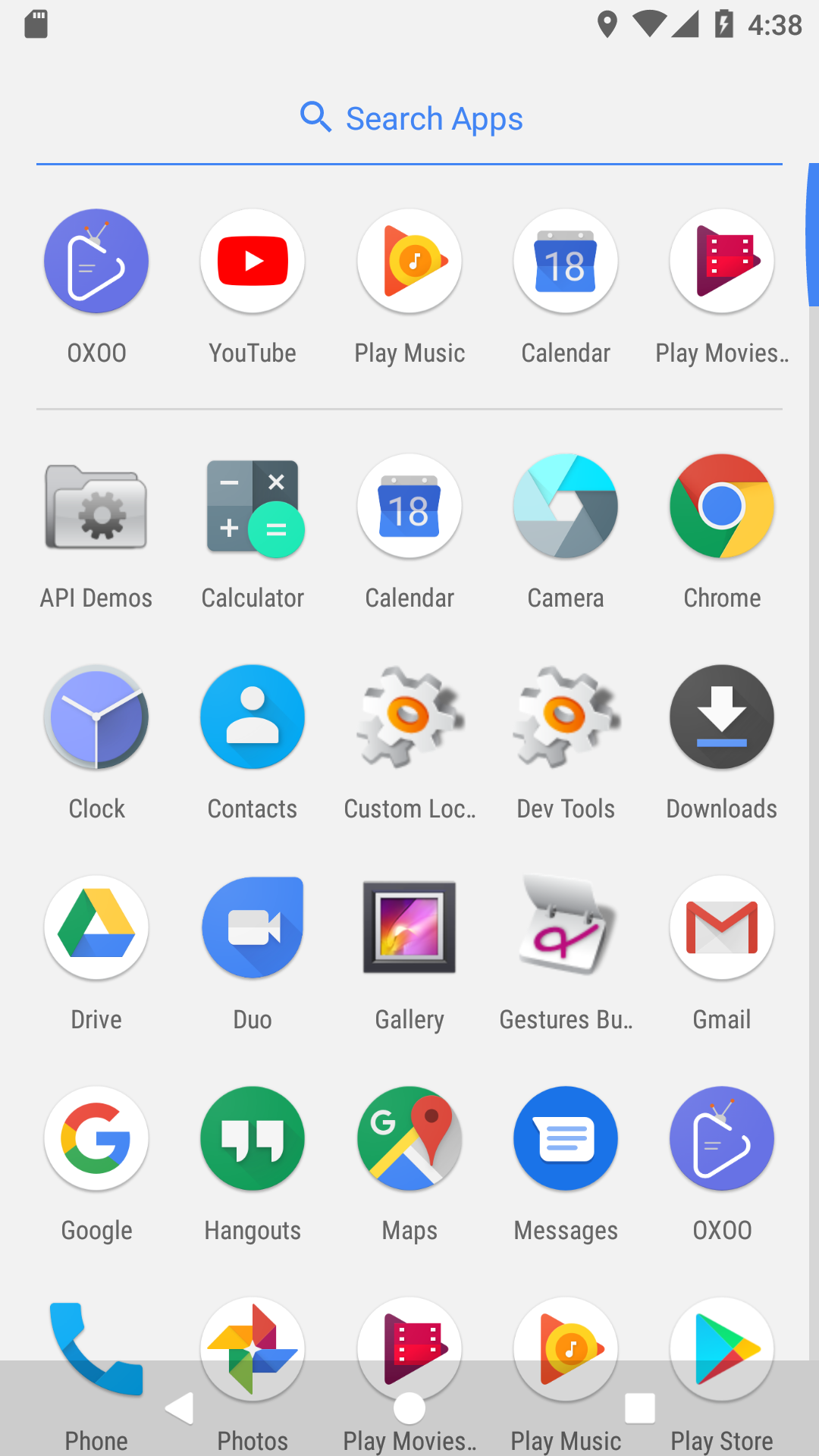The image displays a blurred, grayish background, indicating it was captured from a cell phone screen. At the top, there's a blue magnifying glass icon along with the text "Search apps" written in blue. Directly beneath it is a blue line spanning the width of the screen. The screen is organized into six rows of app icons, each consisting of five icons.

- **First Row:** 
  - OXOO
  - YouTube
  - Play Music
  - Calendar
  - Play Movies

- **Second Row:** 
  - API Demos
  - Calculator
  - Calendar
  - Camera
  - Chrome 

- **Third Row:** 
  - Clock
  - Contacts
  - Custom Lock
  - Dev Tools
  - Downloads

- **Fourth Row:** 
  - Drive
  - Dual
  - Gallery
  - Gesture Buddy
  - Gmail

- **Fifth Row:** 
  - Google
  - Hangouts
  - Maps
  - Messages
  - OXOO 

- **Sixth Row:** 
  - Phone
  - Photos
  - Play Movies
  - Play Music
  - Play Store

Each app icon is clearly visible and neatly arranged, making navigation simple and organized.